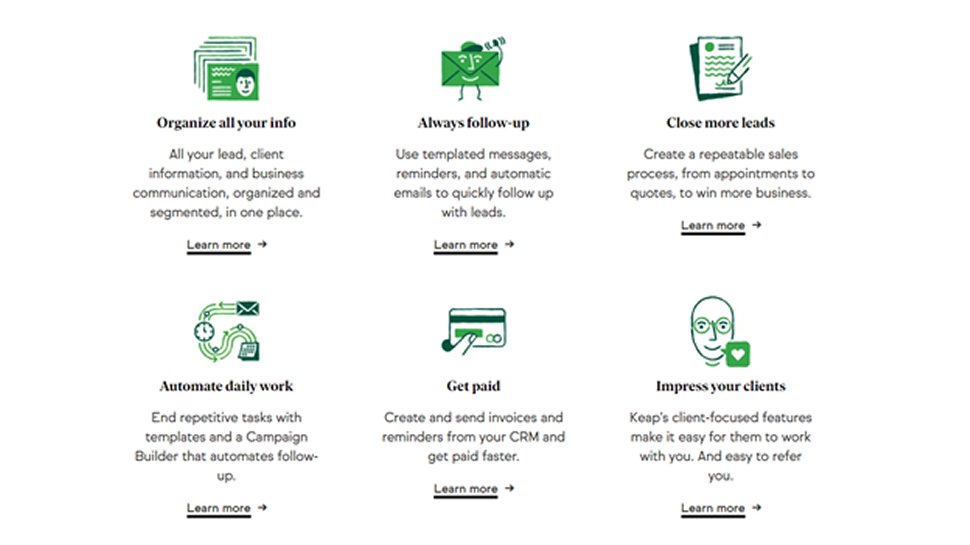The image showcases a structured and detailed representation of six different categories for organizing and enhancing business activities. 

1. **Top Left**: A section titled "Organize All Your Info" features multiple business card icons, with the front card colored green. This segment details how to compile lead client information and business communications in an organized and segmented manner.
   
2. **Below First Section**: A text that reads "All your lead client information and business communication organized and segmented in one place," emphasizing efficient information management.

3. **Middle Left**: Positioned to the right of the first section, the segment titled "Always Follow Up" includes a green envelope emoji. It highlights the use of templated messages, reminders, and automatic emails to facilitate quick follow-ups with leads.

4. **Middle Right**: Adjacent to "Always Follow Up," the section "Close More Leads" is marked with a pencil and paper icon. It explains the process of creating a reputable sales process from appointments to quotes to win more business. Below it, the text describes automating daily work and repetitive tasks with templates and a campaign builder for automated follow-up.

5. **Next to Close More Leads**: The "Get Paid" section emphasizes creating and sending invoices and reminders through your CRM to expedite payments. This section features a credit card icon.

6. **Far Right**: The last category, "Impress Your Clients," includes a sketch of a person’s face within a green square accompanied by a heart icon. This segment discusses keeping clients focused with user-friendly features, making it easier for clients to work with you and refer you.

**Bottom Section**: Below all sections, there is a designated area for learning more about these offerings. The entire layout is set against a clean white background, ensuring clarity and focus on each section's content and icons.

This organized format visually and textually communicates the functionalities and benefits of various business management tools and strategies.